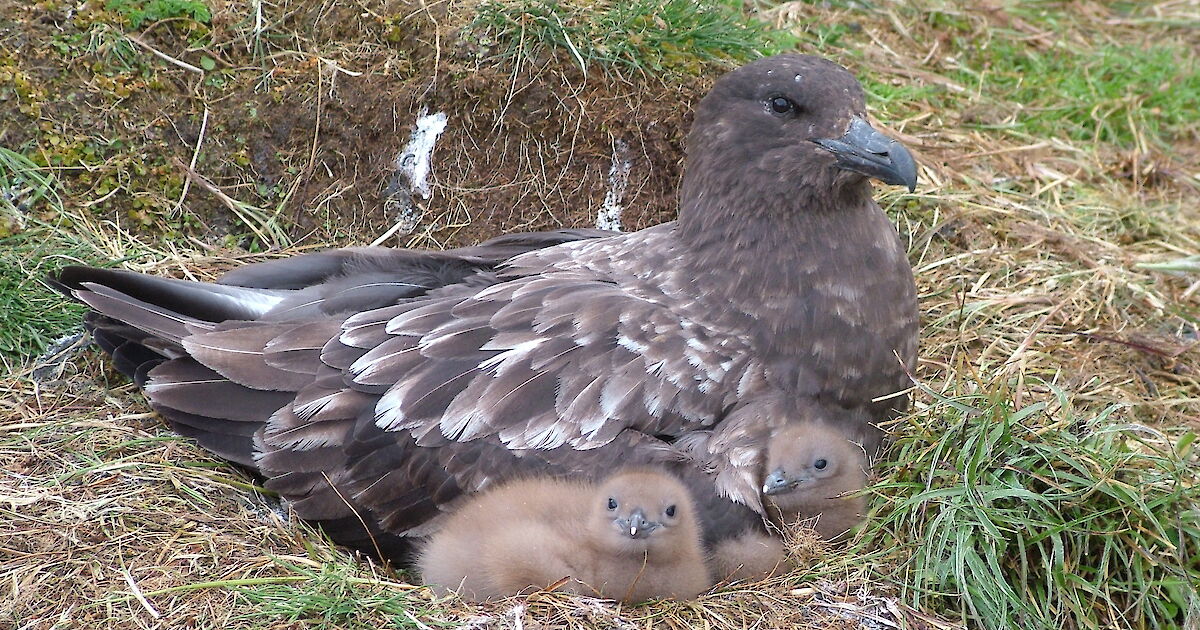In a vibrant, green and brown garden or farm setting, illuminated by daylight, a captivating scene unfolds featuring a majestic bird amidst the grass and patches of sandy soil with occasional twigs and bushes. The bird, which resembles a cross between a goose, pigeon, and hawk, boasts a gray and white plumage with touches of brown on its head, neck, and chest. Its light gray wings with white tips are folded across its back, and it possesses a striking blue beak. The bird is positioned in profile, facing right, but tilts its head slightly upwards as if acknowledging the viewer. Nestled comfortably beneath this bird are two vulnerable chicks with sparse, light purplish down covering their bodies. They possess small beaks and black eyes that gaze out curiously. One chick, centrally located in the image, gazes at the viewer while tucking its tiny claws under its body. The other chick positions itself near the mother, facing its sibling. The realistic, color photograph, captured in landscape orientation, masterfully blends the vivid greenery and dying patches of grass into a picturesque backdrop.